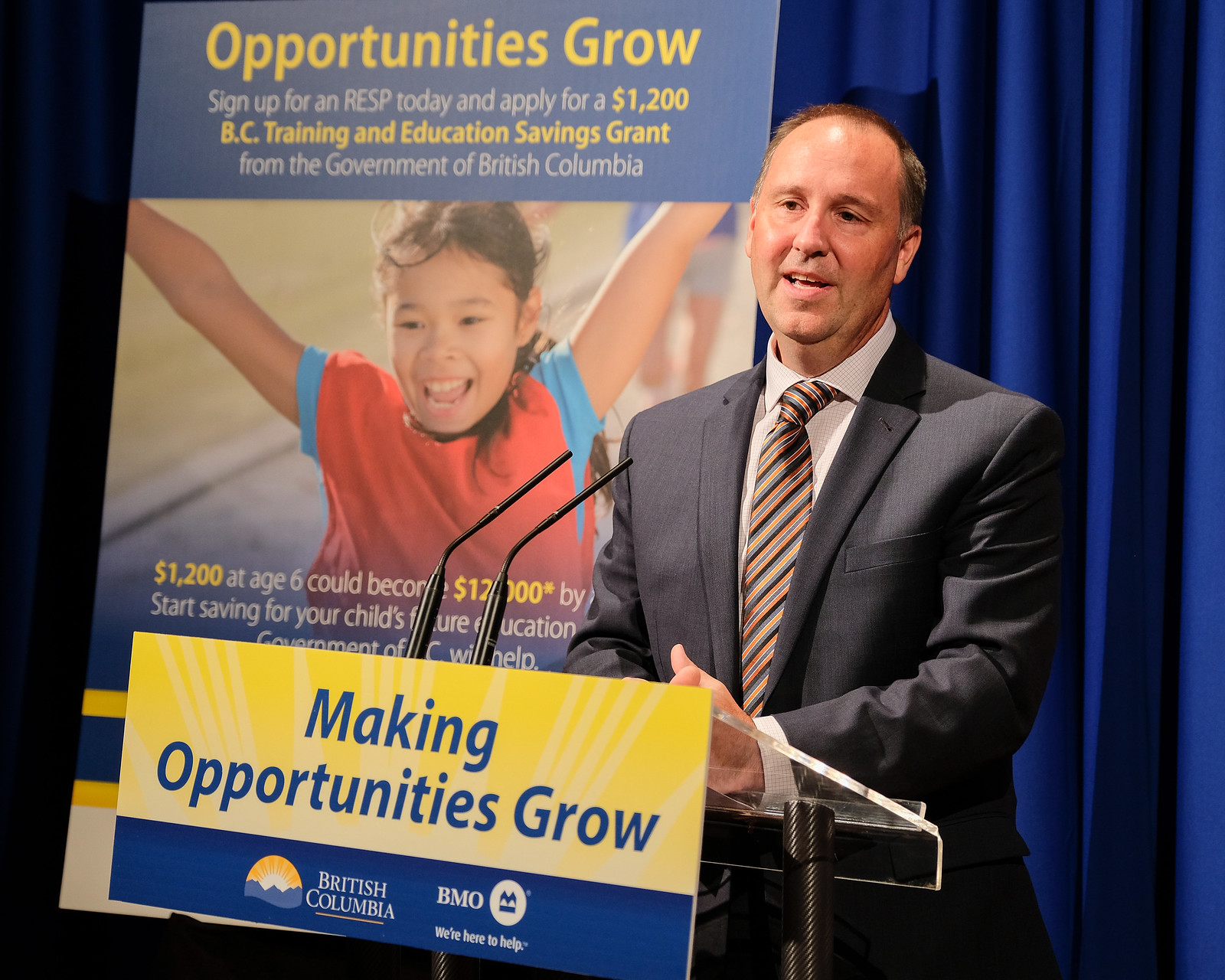The image depicts an older Caucasian man, likely in his 40s or 50s, dressed in a professional black suit with a multi-colored tie (orange, blue, white, and black), standing confidently at a podium mid-speech. The podium is adorned with a yellow and blue sign bearing the phrases "Making Opportunities Grow," "British Columbia," "BMO," and "We're Here to Help." Behind him hangs a navy blue curtain, which conceals the rest of the room. Also visible in the background is a large poster featuring a young, red-shirted Asian girl with blue sleeves. The poster's text encourages viewers to "Sign up for an RESP today and apply for a $1,200 BC Training and Education Savings Grant from the Government of British Columbia." The text highlights that "$1,200 at age 6 can become $120,000," although part of the statement is obscured by the man's arm. Additional messaging, partially visible, advises starting early to save for a child’s future education, emphasizing support from the government of British Columbia.